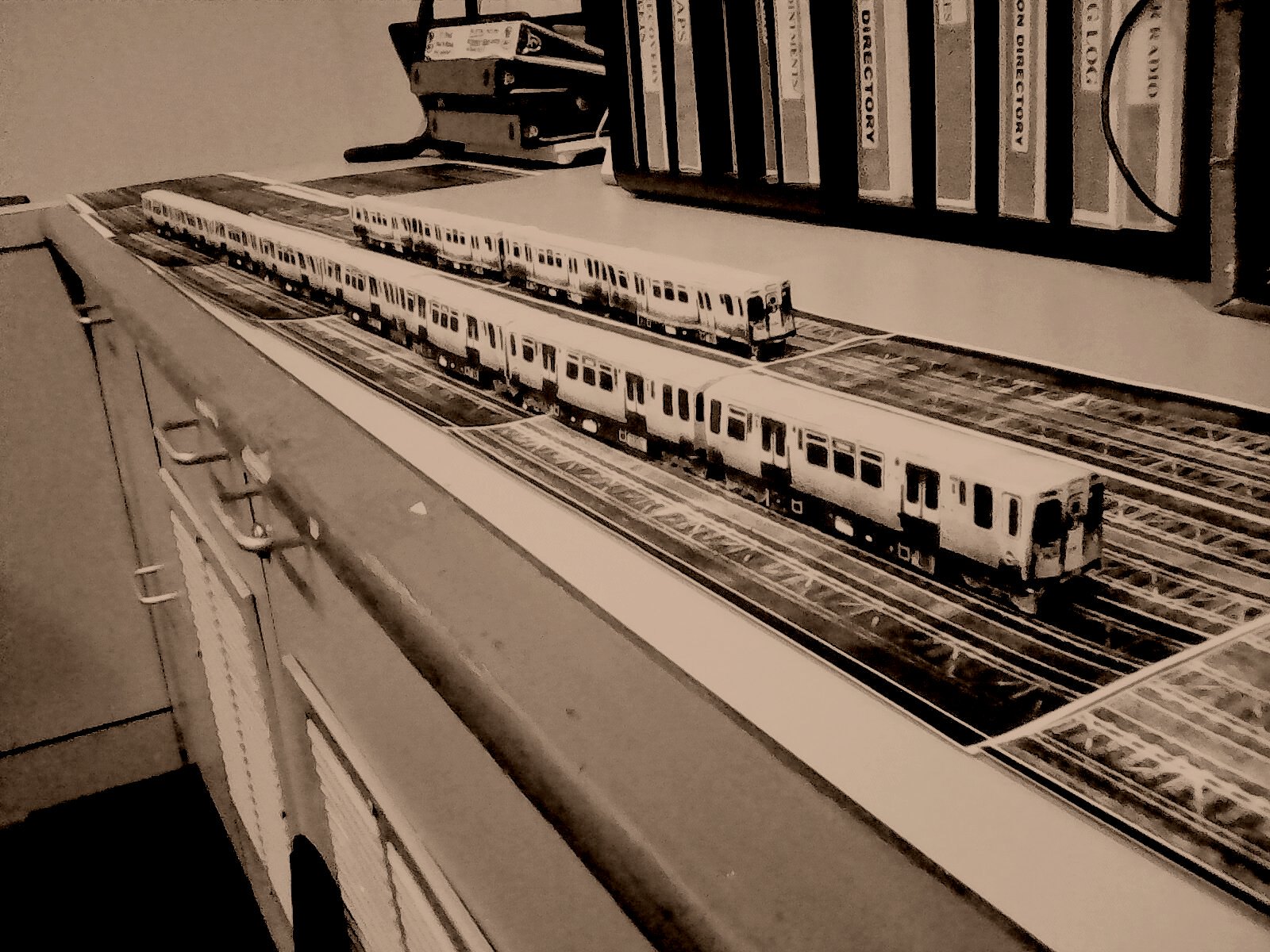The black and white photograph, rendered in a sepia tint, captures an intriguing scene within a lab or office setting. Central to the image is a worktop adorned with a series of long photographs depicting railway tracks. Positioned atop these photographs are detailed model trains; the closest model, potentially a subway train, features five or six carriages, while a smaller model in the background has three or four. These models stretch out along four or five tracks. Beneath the worktop are drawers and doors, suggesting storage space, while above, shelving units house various binders and notebooks. One shelf displays binders upright, while another has them lying on their sides. Some of the binders feature the word "directory." The overall scene is steeped in shades of grey, with the wall in the background appearing light grey, contributing to the vintage and meticulous atmosphere of the image.